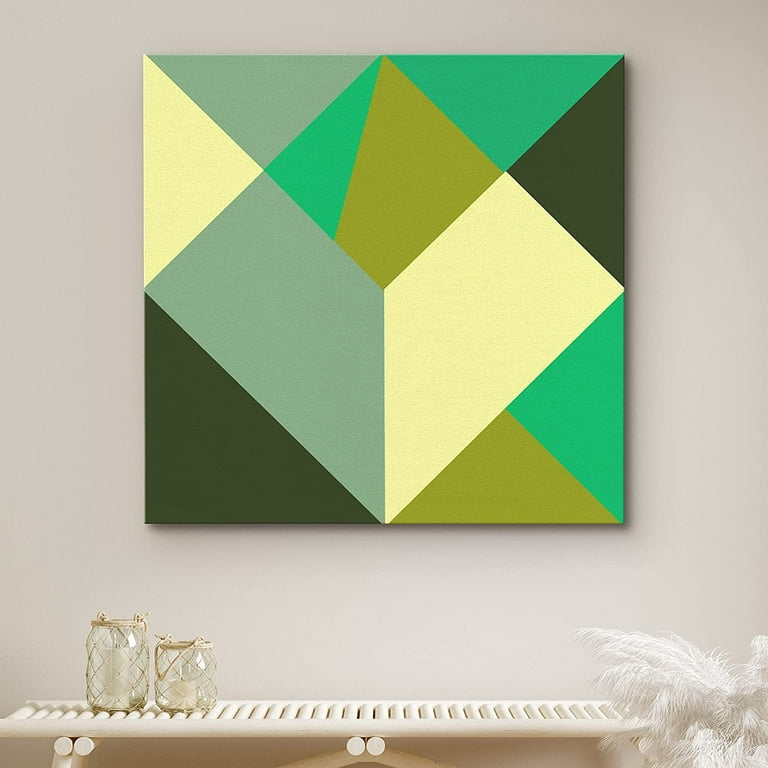The image depicts an abstract painting mounted on a light gray wall. The square-shaped piece features a collection of intricate geometric shapes in various colors. At the top, two inverted triangles are placed, with the left triangle in a grayish-green hue and the right in green. Between them, there's a diamond shape, half green and half mustard green. The lower part of the artwork consists of a solid black section on the bottom left, while the bottom right is split between mustard green and vibrant green.

Below the painting stands a white bench with a louvered design, featuring multiple row patterns. On the left side of the bench are two glass jars with wicker-like lacing around them, which still allow for a clear view inside. The jars, possibly containing candles, add an additional element of interest to the scene. To the right of the jars, white feathers contribute to the overall aesthetic. The setting is brightly lit, making the colors of the painting vivid and the details sharp and easily discernible.